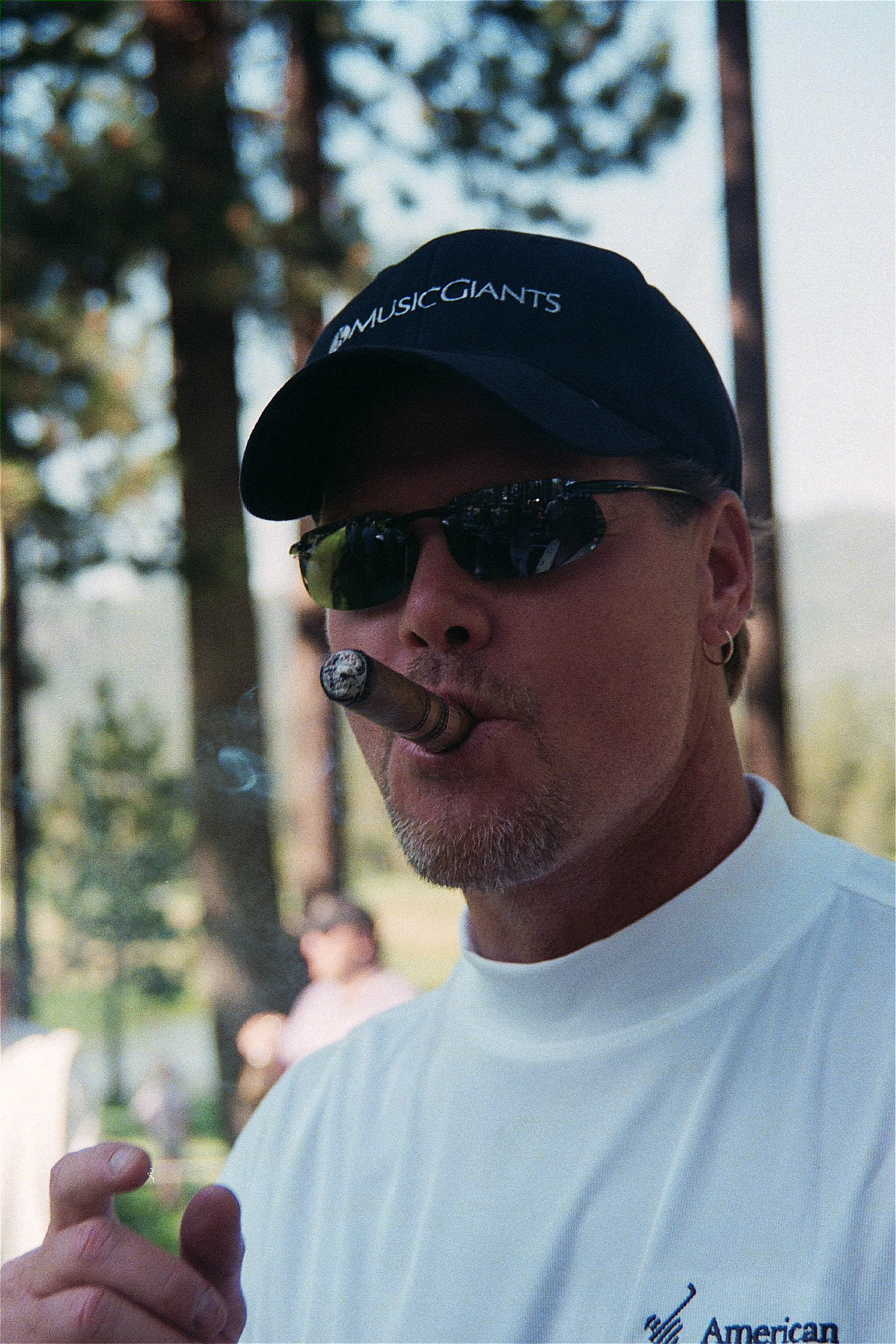This detailed photographic image captures a middle-aged, light-skinned man, possibly in his forties or fifties, outdoors during the daytime. His face appears somewhat reddish and adorned with a thin, stubbly goatee with patches of brown and gray. He wears dark aviator-style sunglasses and has a partially burned cigar in his mouth, his lips puckered around it, with faint smoke rising. A small, thin mustache is visible above his upper lip.

He is dressed in a white t-shirt that features the word "American" in black letters, accompanied by a stylized graphic of a golfer swinging a club on his left chest area. His right hand appears in the bottom-left corner of the image, with fingers bent as if about to pinch something between his thumb and forefinger. On his head, he sports a black baseball cap with the words "Music Giants" embroidered in white above the bill. A small ring-shaped earring can be seen in his left ear.

The background is out of focus but distinctly shows tall trees, possibly pine trees, with green foliage at the top and a clear blue sky with white clouds. There are also mountains visible in the distance. Additionally, a vaguely discernible figure, likely a woman, can be seen in the blurry background, appearing to wear a white shirt and possibly a dark hat. The scene conveys a casual, relaxed moment amidst a scenic outdoor setting.